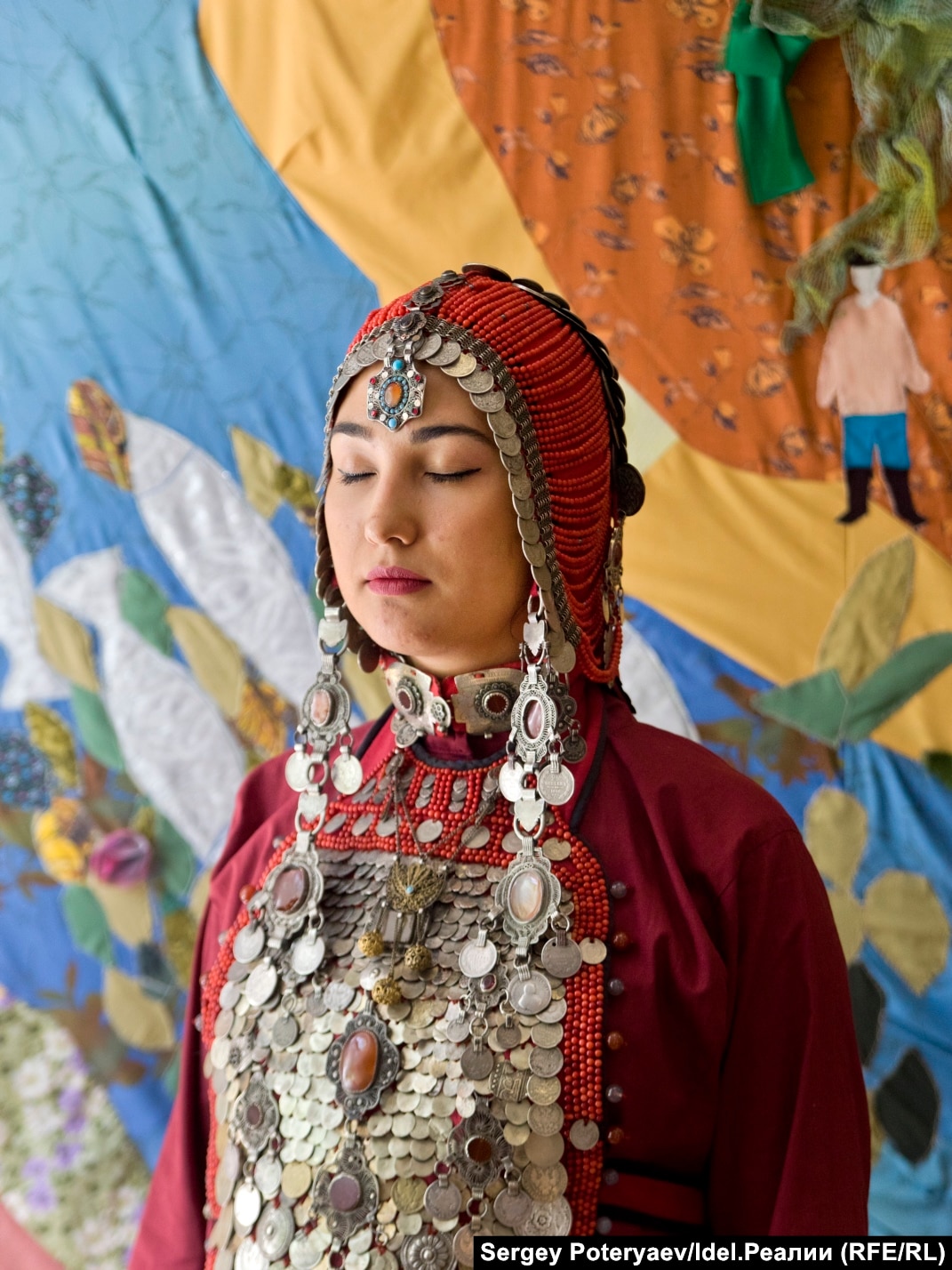In this color photograph, a woman with closed eyes stands solemnly, perhaps in prayer, adorned in traditional, ceremonial attire. She wears a maroon head covering richly decorated with metal discs that resemble coins, red beads, and assorted jewels. Dangling long silver earrings frame her face, accentuating her dark eyebrows and long black eyelashes. A distinctive gold, aqua blue, and orange pendant hangs over her forehead. Her outfit, a cranberry-colored suit, includes a loose, long-sleeved top with a beaded bib or apron fashioned from red beads and additional silver-like discs. The scene is set against a fabric backdrop, possibly a handmade quilt or tapestry, showcasing vibrant colors—blue, white, yellow, and orange—and floral patterns along with a stitched image of a man. In the bottom part of the image, a black rectangle features white text stating "Sergey Poteryaev / ldel.pea" followed by Cyrillic characters and "(RFE/RL)," suggesting the photographer's name and affiliations.